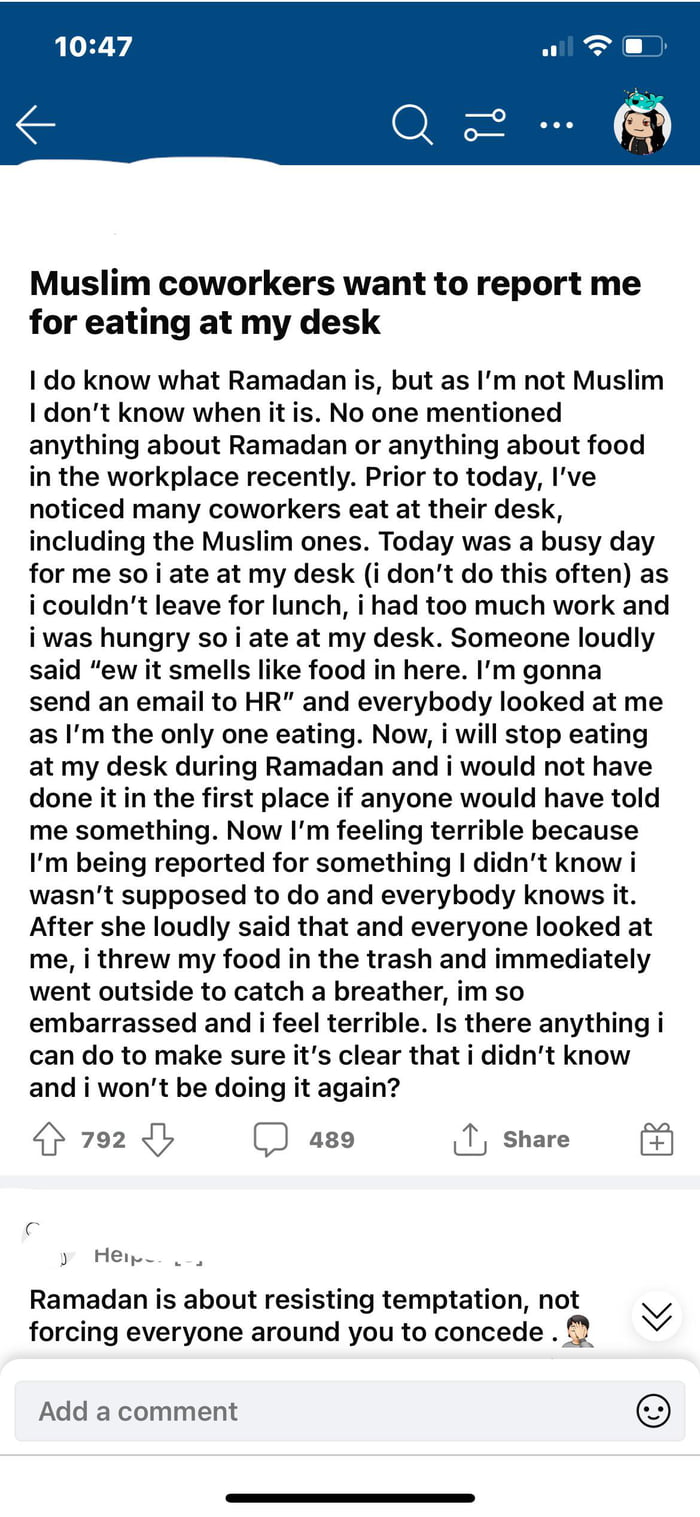This screenshot captures a section of a Reddit post with notable edits and markers. The image prominently features the Reddit app interface with a white background. In the top right corner, you can see the user's Reddit profile photo. Key information such as the post author's username, profile picture, and the name of the subreddit has been obscured using white paint. The title of the post, written in large, bold black letters, stands out at the top.

Directly beneath the title is the lengthily composed body of the post, barely visible in the screenshot due to its extensive length. At the bottom of the post, Reddit's typical interaction icons are present: an upward arrow for upvoting, a downward arrow for downvoting, and in between these is the number 792, indicating the post's current upvote count. Next to these icons, a chat bubble icon shows that there are 489 replies to the post. To the right of the chat bubble is a share icon.

Below this primary post information, there's a brief one-sentence reply from another user, though their information has also been edited out with white paint. At the screenshot's very bottom, an "Add Comment" bar is displayed, with a small smiley face emoji located on the far right of this bar.